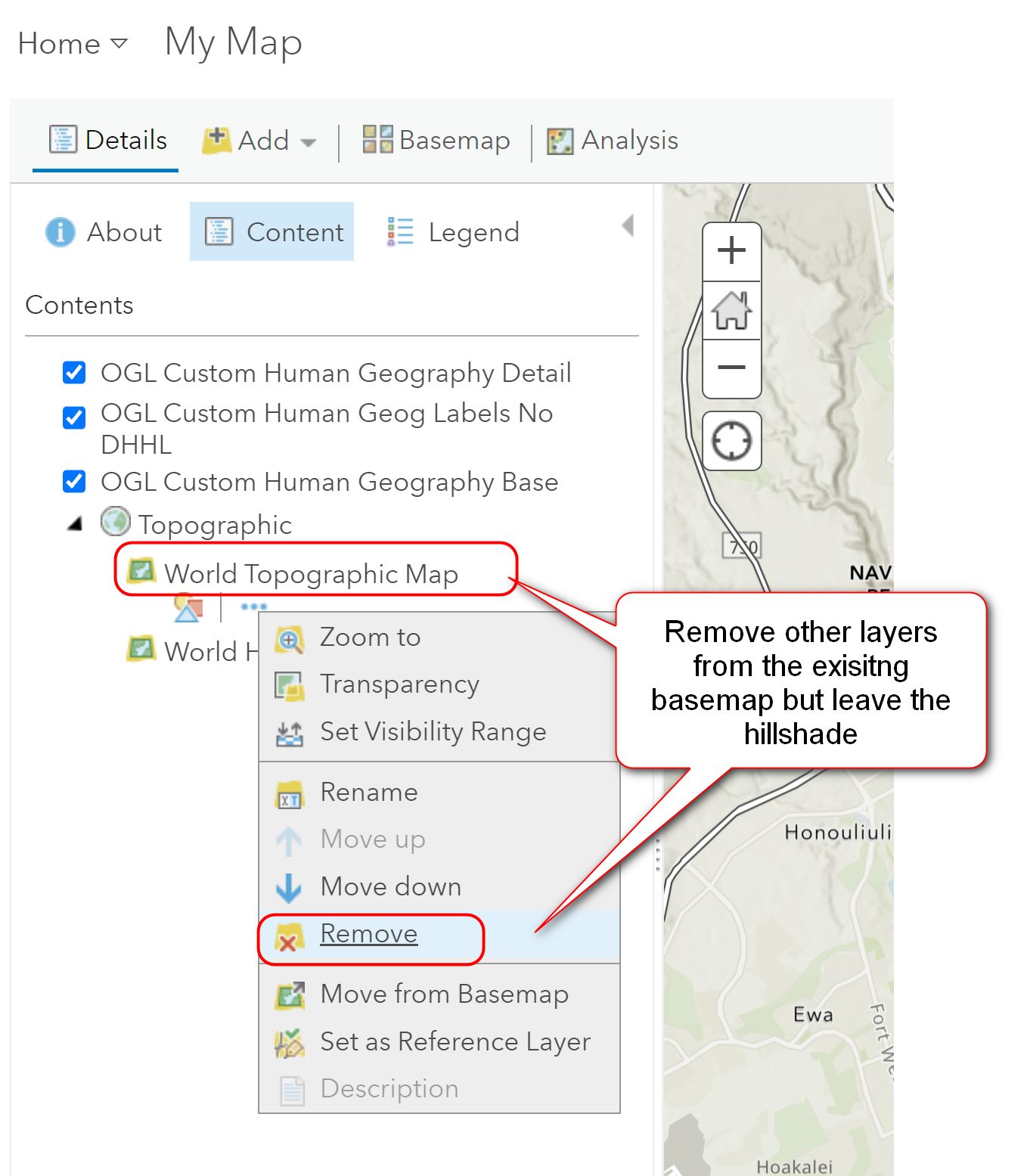This detailed descriptive caption provides a comprehensive overview of the screenshot:

"The screenshot captures an interface of an unidentified website, focusing on a detailed map and navigation panel. At the top of the interface, a menu bar displays several options, including 'Home,' 'My Map,' 'Details' (currently selected), 'Add,' 'Base Map,' 'Analysis,' 'About,' 'Content' (also selected), 'Legend,' and 'Contents.' Within the 'Contents' section, several layers are listed: 'OGL Custom Human Geography Detail' (selected), 'OGL Custom Human Geography Labels' (unselected), 'No DHHL' (selected), and 'OGL Custom Human Geography Base' (selected). Below these options, the term 'Topographic' and 'World Topographic Map' are highlighted within a red rectangle. A pop-up window appears on the interface, showcasing options like 'Zoom To,' 'Transparency,' 'Set Visibility Range,' 'Rename,' 'Move Up,' 'Move Down,' 'Remove,' 'Move from Base Map,' and 'Set as Reference Layer Description.'

To the right, a map of an unidentified area is partially visible. Superimposed on the map is a white rectangle with arrows pointing to the 'World Topographic Map' and 'Remove' buttons. Inside this white rectangle, text reads: 'Remove Other Layers from the Existing Base Map, but Leave the Hill Shade.' The screenshot distinctly lacks any human presence or additional contextual details."